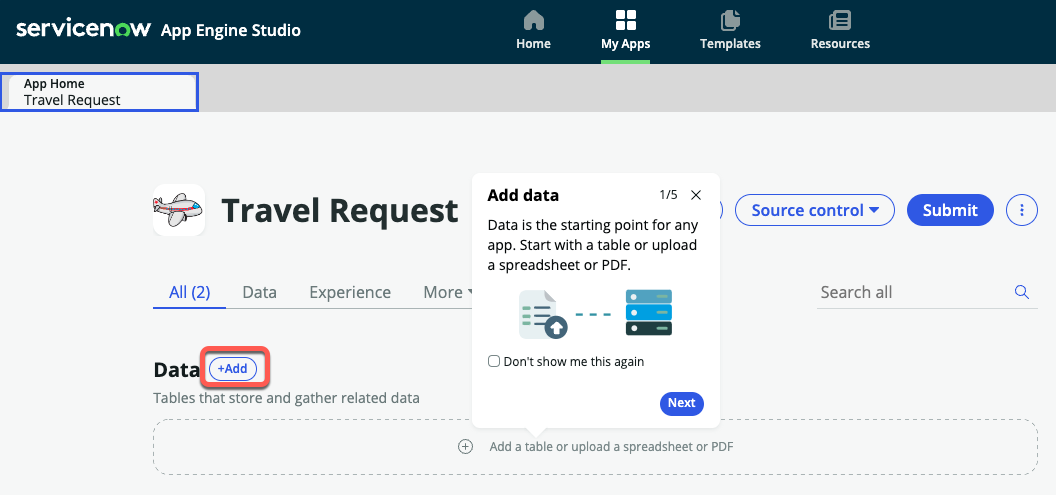The image is a screenshot from a ServiceNow web page, specifically from the App Engine Studio interface.

At the top of the page, there is a dark gray header with all text displayed in white. On the left side, the ServiceNow logo is prominently featured. The logo is in a lowercase font, with "ServiceNow" as one word. Notably, the "O" in "now" is uniquely colored green. To the right of the logo, the header reads "App Engine Studio."

On the menu bar, which spans from the center to the right, we see several navigation options. From left to right, these include: a home icon followed by the word "Home," a section labeled "My Apps" with an accompanying icon of four white squares above it, "Templates," and "Resources." The "My Apps" section is highlighted, indicating it has been selected.

Beneath the menu, there is a light gray border. Within this border, on the left side, is a white rectangle containing the text "App Home Travel Request." The rest of the page has a white background.

To the left, in large bold font, the words "Travel Request" are displayed alongside a small gray airplane icon. 

In the center of the page, there is a white rectangle titled "Add Data" in bold at the top left corner. On the top right corner, the text reads "1/5," next to an "X" icon. Below the title, there is a paragraph explaining that data is the starting point for any app, suggesting options to start with a table, upload a spreadsheet, or upload a PDF. An illustration of a document within a blue circle with an upward-pointing white arrow is next to this paragraph. To the right of the illustration, there are three small rectangles in different colors: grayish-blue, mid-sky blue, and black.

Below this, in gray font, it says "Don't Show Me This Again," next to a checkbox for selecting this option. At the lower right corner of the rectangle, there is a button labeled "Next."